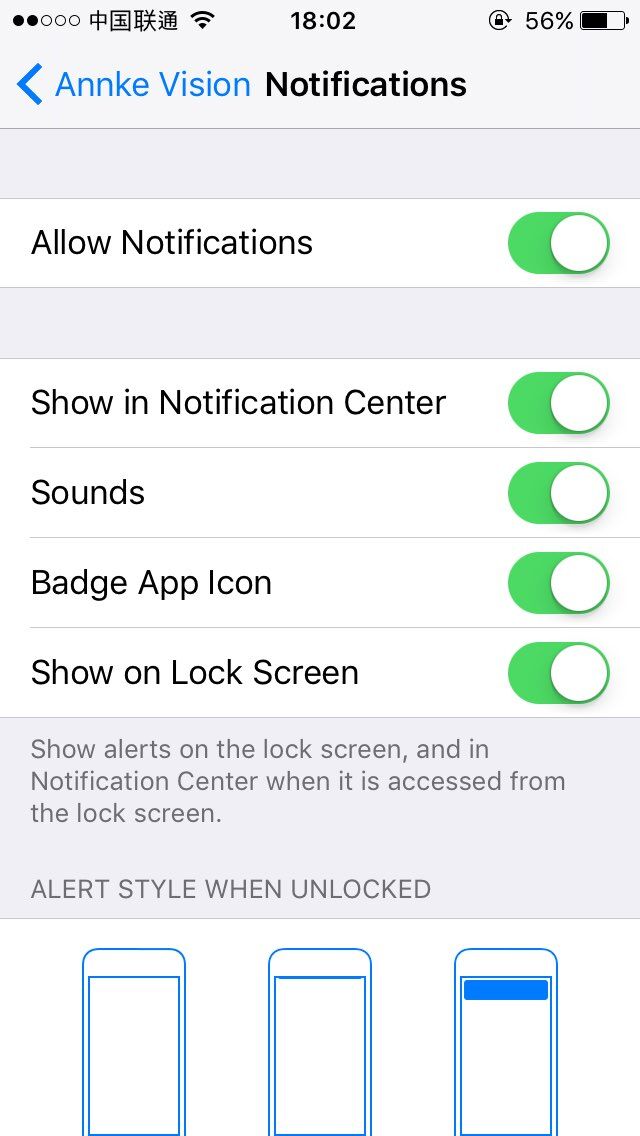This image is a screenshot of a cell phone displaying notification settings for the Anki Vision app. 

In the top left corner, there is a blue arrow pointing to the right, followed by the text "Anki Vision" in blue. Centrally positioned, "Notifications" is shown in bold black letters. 

Descending from there, the settings are listed as follows:

1. Allow Notifications: The toggle switch on the right is turned on.
2. Show in Notification Center: This option is turned on.
3. Sounds: The toggle switch for sounds is enabled.
4. Badge App Icon: This notification feature is turned on.
5. Show on Lock Screen: This option is enabled as well.

Further down, there is a large, light gray, horizontal rectangular box with instructions. It states: "Show alerts on the lock screen and in Notification Center when it is accessed from the lock screen. Alert Style When Unlocked."

On the bottom left of this rectangular box is an image of a cell phone with a light border. In the middle, there is another cell phone image with a darker border, and on the right side is a third cell phone image also with a darker border. A horizontal blue rectangular bar is depicted on the top of the third cell phone image.